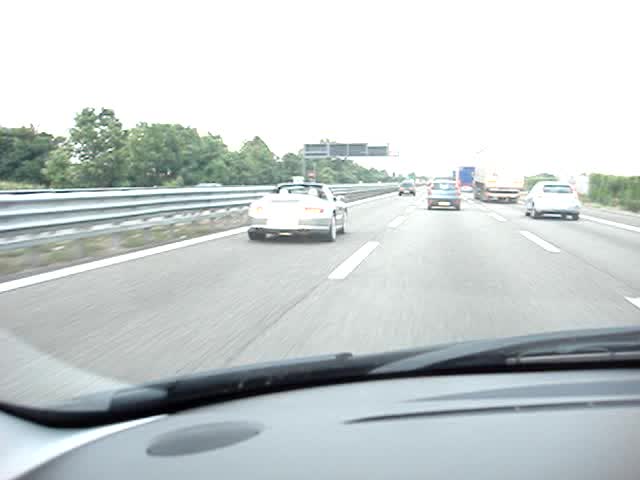This image, captured from the front mirror or possibly the dashboard of a car on the Jarbridge side, showcases an older, slightly overexposed photograph of a three-lane freeway. The perspective appears to be from the driver’s point of view, with part of the dashboard visible at the bottom, including an unused black windshield wiper. The sky is a clear, bright white, suggesting overcast conditions. 

In the left lane, there's a silver convertible, while the middle lane, where the camera vehicle is positioned, has an SUV directly ahead. The right lane features a distant, large truck trailer. More vehicles, including a blue sedan, can also be seen scattered across the lanes. The lanes are demarcated by dashed white lines, and there are barriers along the freeway's sides. Green trees and shrubs line both sides of the highway, adding to the scene's natural backdrop.